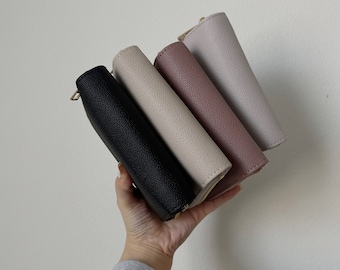In the photograph, a white hand, possibly belonging to a person wearing a blue or gray shirt, is outstretched from the bottom of the frame, delicately holding four rectangular wallets. These wallets, which vary in color—black, tan, pink, and grayish-white—feature thick seams and zippers for closure. All of the wallets appear robust and slightly larger than the hand itself, yet they are expertly balanced at the edges. The monochromatic background, depicted in shades of white or gray, contrasts with the vivid colors of the wallets.